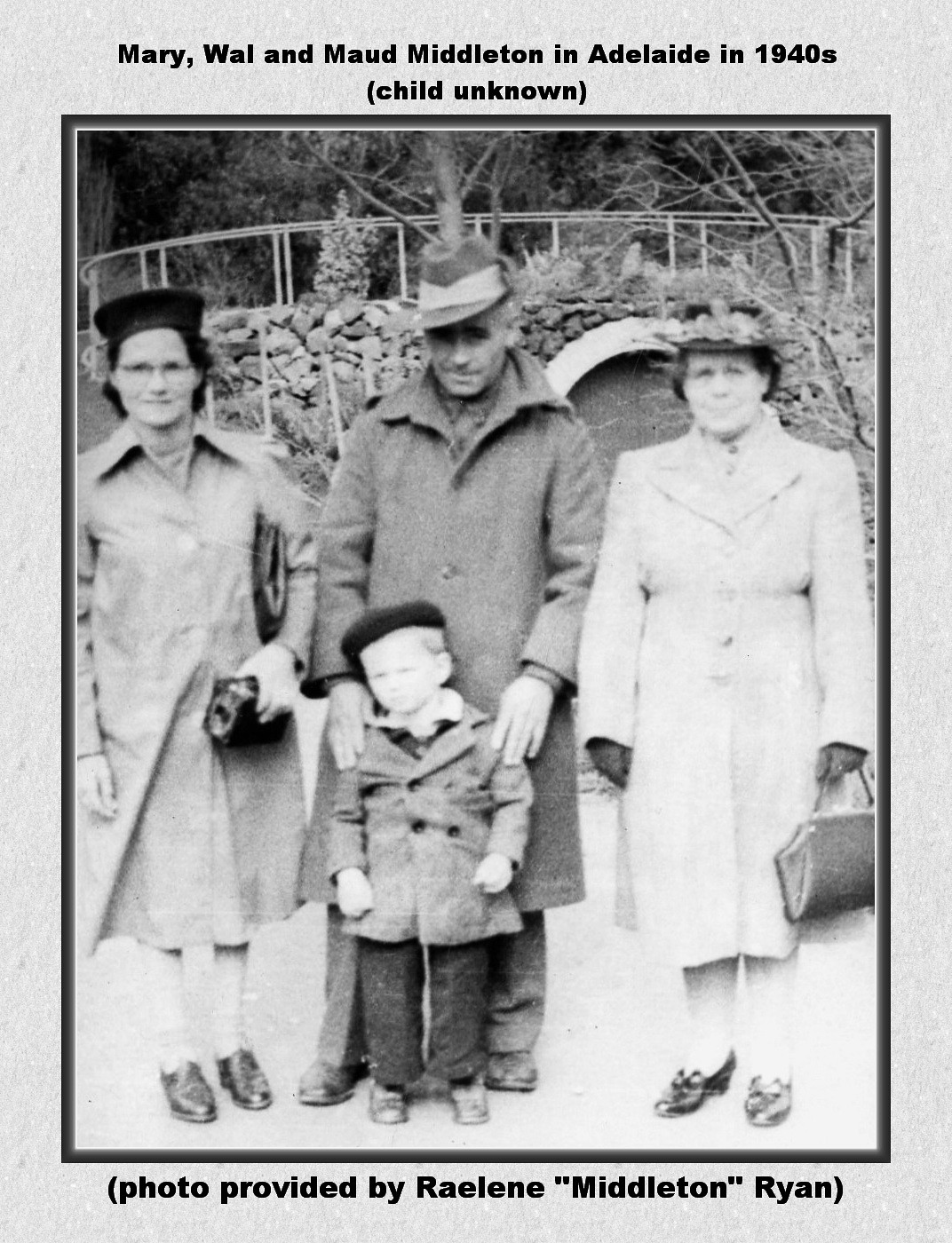Set against a grainy gray backdrop, this old-fashioned black-and-white photograph captures a poignant moment from the 1940s in Adelaide. The image features three adults and one child posed outdoors amidst rugged terrain of rocks and trees. Centered is a man with a hat, gently resting his hands on the shoulders of a small, unidentified boy standing in front of him, also wearing a hat. Flanking the man are two older women, Mary Wall on the left and Maude Middleton on the right, both adorned in long overcoats and hats, each holding a purse. The photograph, slightly blurry, is framed by a faint dark gradient that transitions to a lighter inner border. Text at the top reads, “Mary Wall and Maude Middleton in Adelaide in the 1940s, child unknown,” while the bottom text credits the photo to Raylene Middleton Ryan.